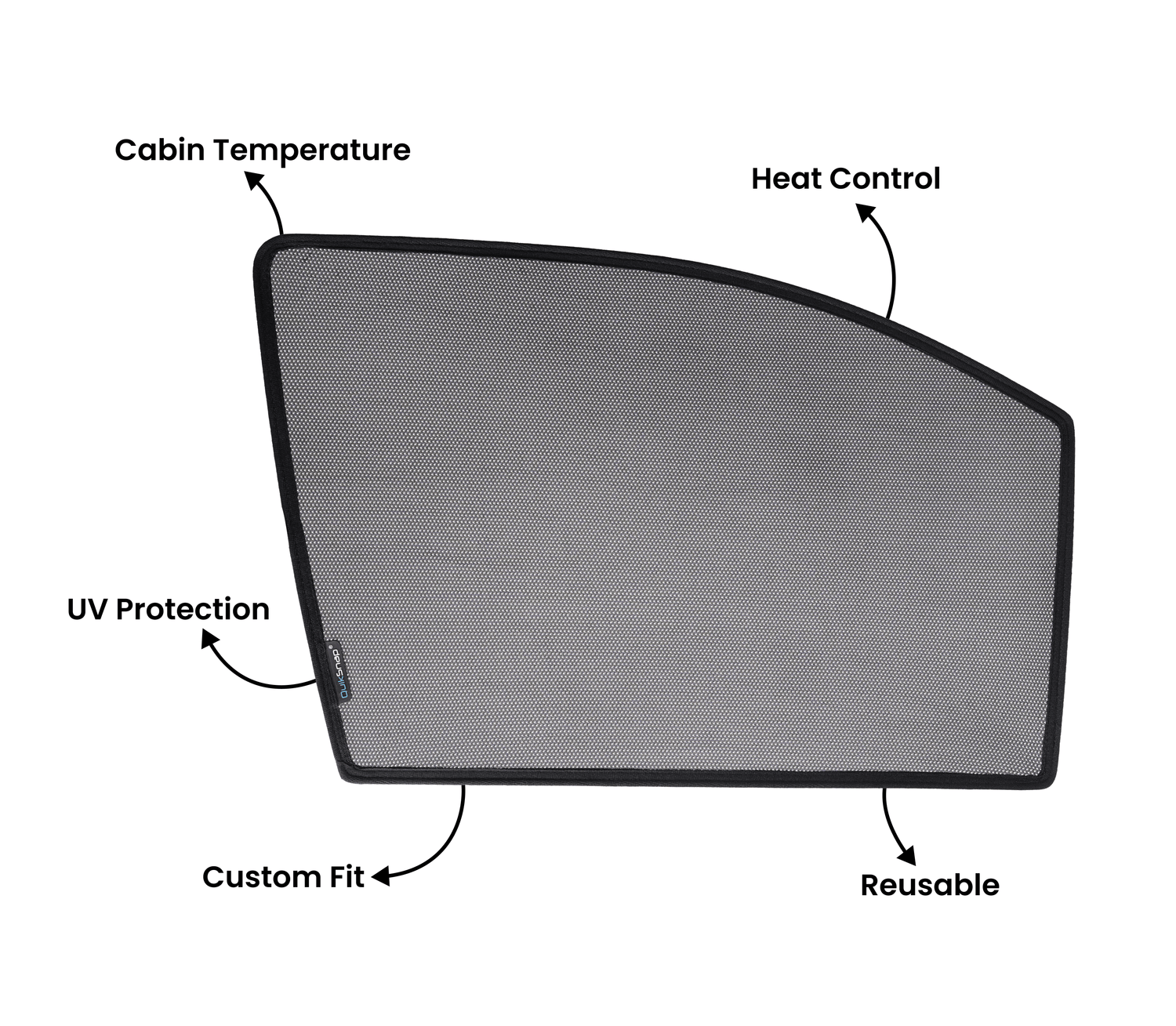The image depicts a window cover or sunshade designed for vehicles, characterized by a gray mesh interior encased in a thick black border. The cover appears rectangular but is slightly elevated on the left side. The background of the image is white, and several black arrows extend from the sunshade, each pointing to bold black text that highlights its features: cabin temperature, heat control, UV protection, custom fit, and reusable. Additionally, there is a small tag on the left side of the sunshade with illegible text in blue and white on a black background.